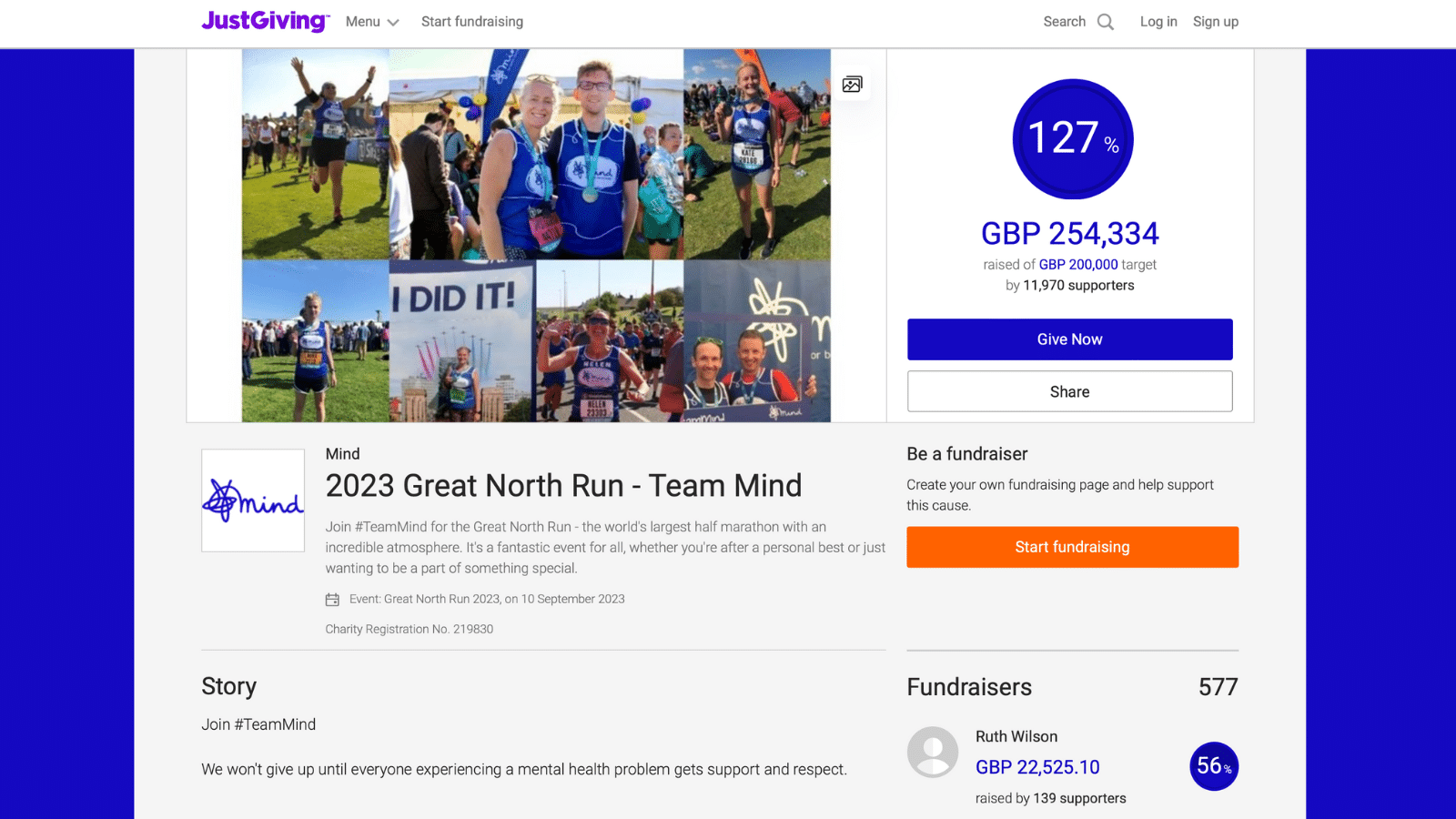In this image, the header displays the JustGiving logo, a trademark symbol (TM), and menu options including "Start Fundraising." On the top right, there are buttons for "Search," "Login," and "Sign Up." The progress bar shows that 127% of the fundraising goal has been reached, with £254,334 raised from a £200,000 target, supported by 11,970 contributors. There are also buttons for "Give Now" and "Share."

Prominently featured is the logo and name of the charity, Mind, under the title "2023 Great North Run." This text encourages individuals to join Team Mind for the Great North Run, described as the world's largest half marathon, celebrated for its incredible atmosphere. The event is touted as fantastic for all participants, whether aiming for a personal record or simply wanting to be part of something special. 

Additional details specify the event as the Great North Run, scheduled for 10th September 2023. Mind's charity registration number, 219830, is included. The caption also shares a motivational story urging potential participants to join Team Mind, emphasizing the charity's commitment to not giving up until everyone experiencing a mental health problem receives support and respect.